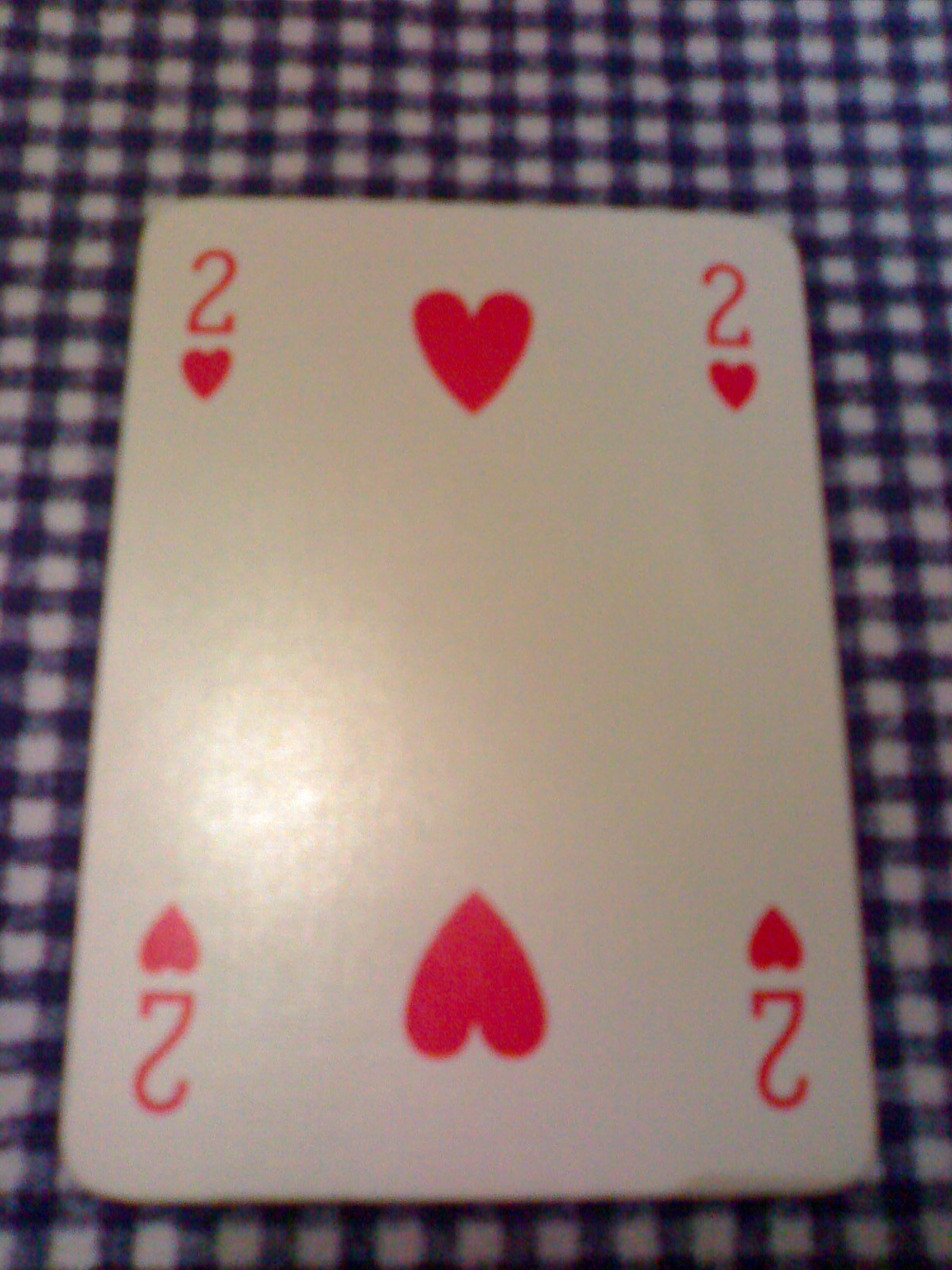This detailed photograph captures a close-up image of a worn and slightly stained two of hearts playing card. The card, which has seen better days, features a number "2" in each corner accompanied by a small red heart underneath each number. The top corners have both numbers and hearts oriented right-side-up, while the bottom corners feature these elements upside-down. Centrally on the card, two larger red hearts are mirrored. The card is positioned on a tablecloth that exhibits a blue and white gingham pattern with hints of red threading through it. This vividly detailed scene is set in an indoor environment, with a subtle glare on the card hinting at a nearby light source.